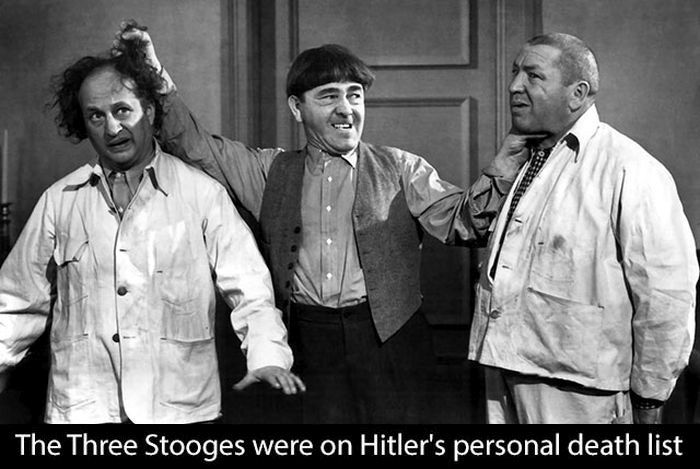In this black-and-white image, the focus is on the three Stooges, arranged from left to right. The Stooge on the left is balding with long hair on the sides and wears a white jacket with three buttons. His expression is one of distress as the middle Stooge, who has an aggressive bowl haircut and dons a gray vest over a dress-down shirt with black pants, mischievously lifts the first Stooge's hair while also placing his other hand around the neck of the Stooge on the right. The middle Stooge's antics bring a silly grimace to his face. The Stooge on the far right is heavier set and bald, wearing lighter colored pants and a checkered shirt under a light jacket. He looks discomforted by the hand under his chin. The backdrop reveals a bare room with a single candle and a closed door visible, which centers the image. The caption beneath the trio is displayed in white text on a black bar, stating, "The three Stooges were on Hitler's personal death list." This image is likely from a nostalgic TV show and could be interpreted as a meme due to its historical and humorous layers.